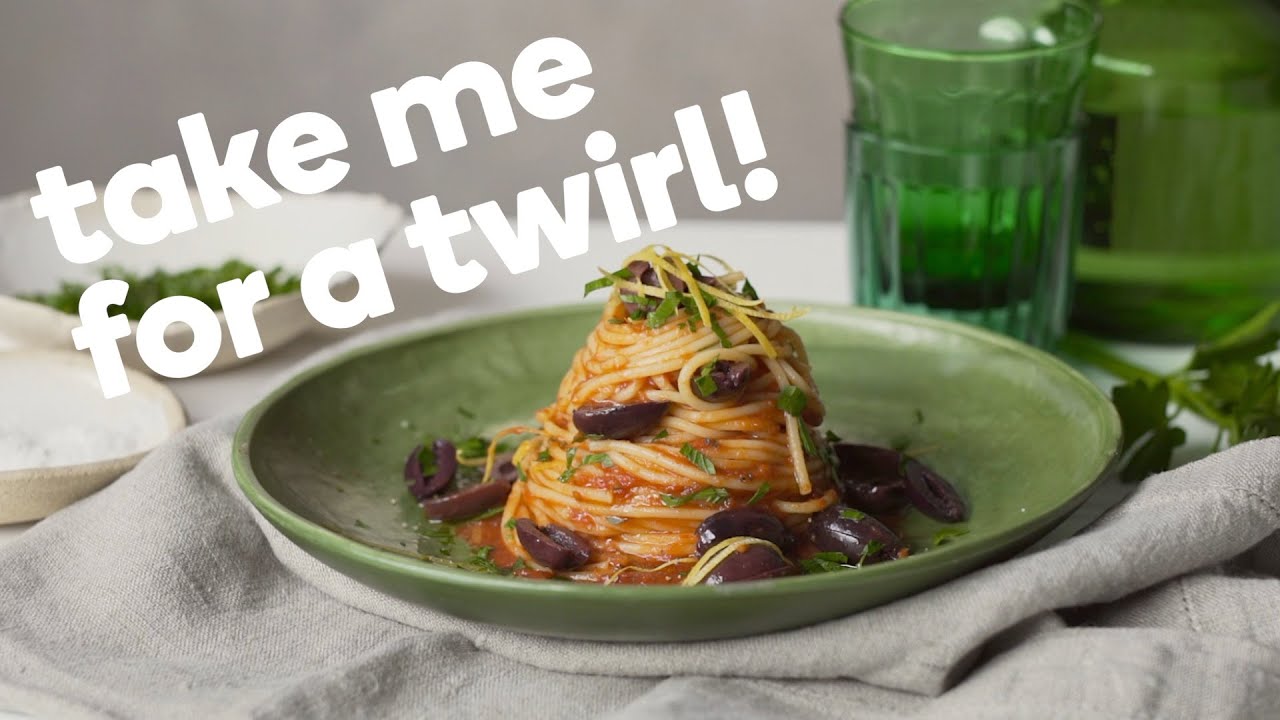In the photograph, a vibrant green circular plate sits atop a light gray, partially folded tablecloth or napkin. Centered on the plate is an impressive, conical mound of spaghetti, neatly assembled to resemble a spiraling volcano. Dressed in a rich red sauce, the spaghetti is garnished liberally with fresh parsley and interspersed with dark brown, halved olives, adding a touch of earthy color both on top and around the base of the pasta.

In the background on the right-hand side of the image, a green drinking glass, possibly accompanied by a green jug, adds a refreshing contrast. On the upper left of the picture, bold white, lowercase letters spell out, "take me for a twirl!", inviting engagement with the enticing dish. The backdrop features a gray wall, complementing the overall color scheme. Additionally, in the background on the left side, two white dishes can be observed. One dish appears to contain green herbs, further harmonizing with the vibrant plate and the theme of fresh ingredients.